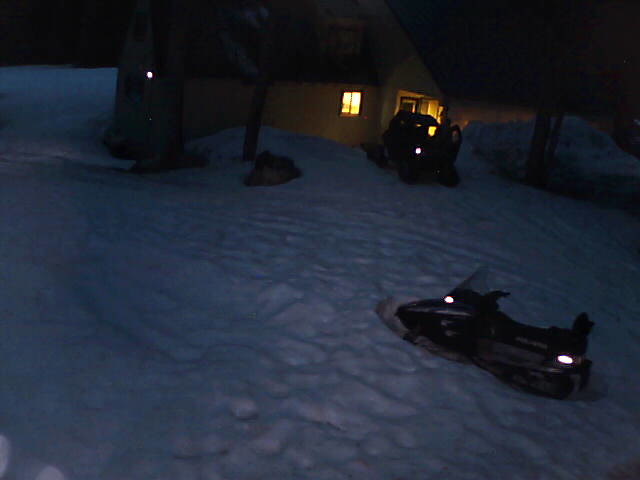This night-time photograph captures an isolated small house, possibly yellow or tan, nestled in a snowy forest. The snow is deeply accumulated, with high piles plowed to the right of the house and numerous footprints marking the trampled surface around it. The snow, tinged with a hue of blue due to the dark conditions, reflects the soft yellowish and white lights emanating from the windows and the fluorescent lighting inside the house. 

In front of the house, near the entrance, a small vehicle, possibly a quad, is parked with its rear lights on. Nearby, a snowmobile, parked sideways with the lights still on, stands partly obscured in the deep snow, its tracks visible in the background. The house has a brown roof and a possible second story or an attic window. The surrounding forest trees frame the scene, adding to the serene yet solitary ambiance of this snowy woodland retreat.